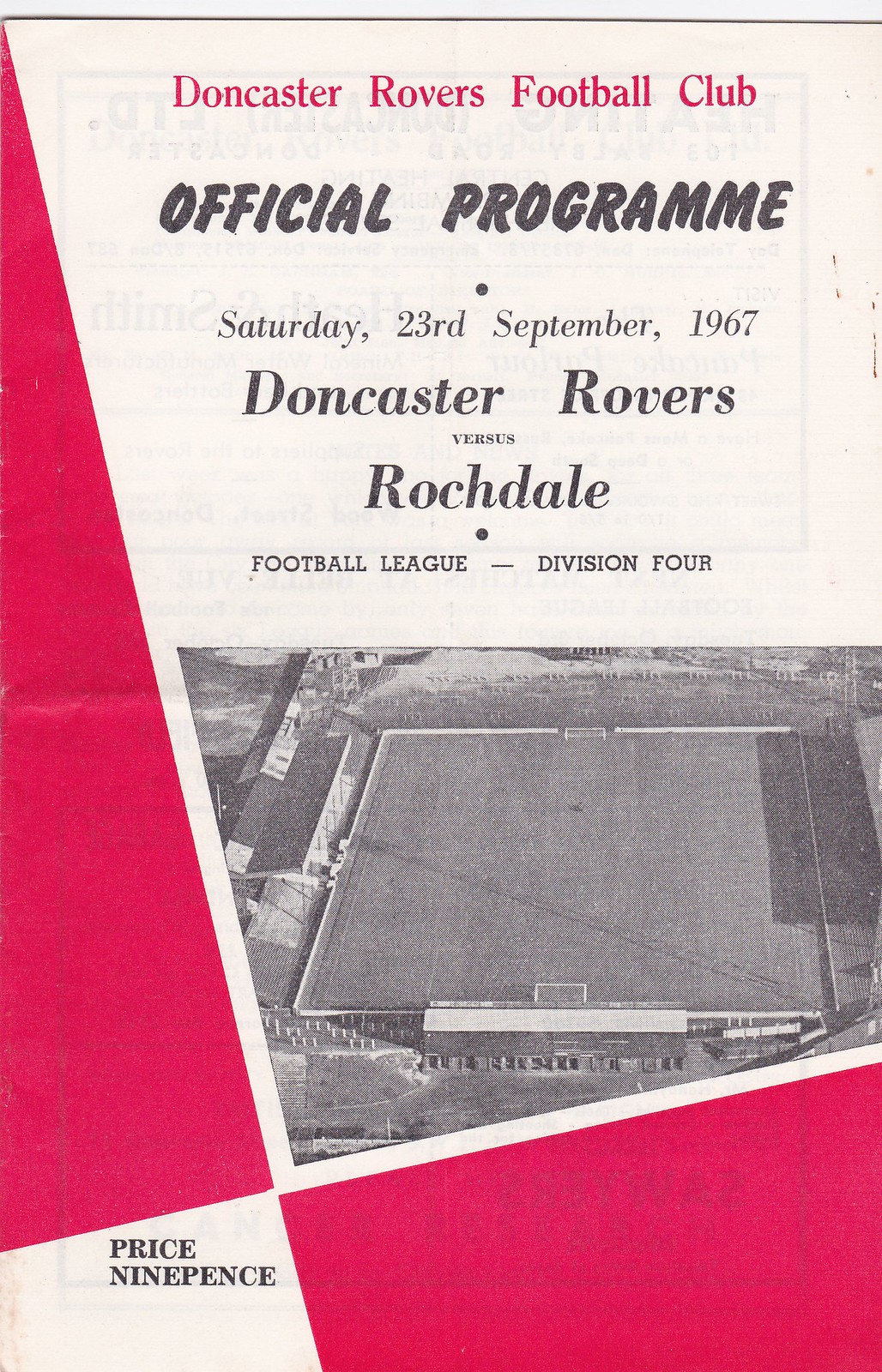The image depicts the cover of an official program for the Doncaster Rovers Football Club, dating Saturday, 23rd September 1967. The design prominently features a white background embellished with bold red triangles and rectangles. At the top, bold red text announces "Doncaster Rovers Football Club," with "Official Program" in black letters just below it. Further down, the date "Saturday, 23rd September 1967" is listed, followed by the match details "Doncaster Rovers vs. Rochdale," specifying it as a Football League Division 4 game.

Beneath the textual information, a grainy black-and-white photograph offers an aerial view of the football field, capturing the stands and the sparsely grassed, somewhat neglected playing surface characteristic of the era. The thin, aged paper of the program reveals faint impressions of articles from the reverse side. Decorative red geometric shapes adorn the lower section of the cover, adding visual interest to the vintage design. In the bottom left corner, the cover notes the price of nine pence.